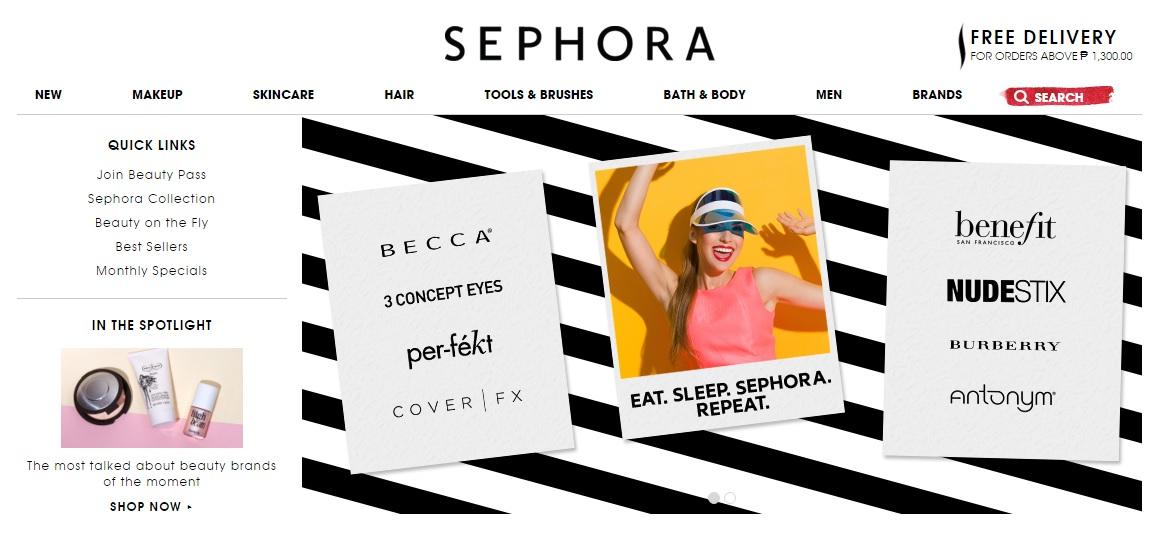The image showcases the homepage of the Sephora website. At the top, the prominent Sephora logo is displayed, with a right-hand sidebar announcing free delivery for orders exceeding a certain amount. Directly beneath this announcement, a horizontal menu features categories such as New, Makeup, Skincare, Hair, Tools & Brushes, Bath & Body, Men, Brands, and a Search function. The Search option stands out in red with an accompanying icon.

To the left, there’s a Quick Link section offering direct access to Join Beauty Pass, Sephora Collection, Beauty on the Fly, Best Sellers, and Monthly Specials. A fine grey line separates this from another section labeled "In the Spotlight," which includes a small image of products and a "Shop Now" link.

The main content panel on the right displays three white rectangles against a stylish black-and-white patterned background. Each rectangle contains text and images: 
1. The first rectangle highlights "Becca, 3 Concept Eyes."
2. The second features a smiling girl with text reading "Eat, Sleep, Sephora, Repeat."
3. The third advertises brands like Benefit, Ude, STX, Burberry, and Antonym, listing product names.

Overall, the homepage balances vibrant visuals with user-friendly navigation and promotional highlights.